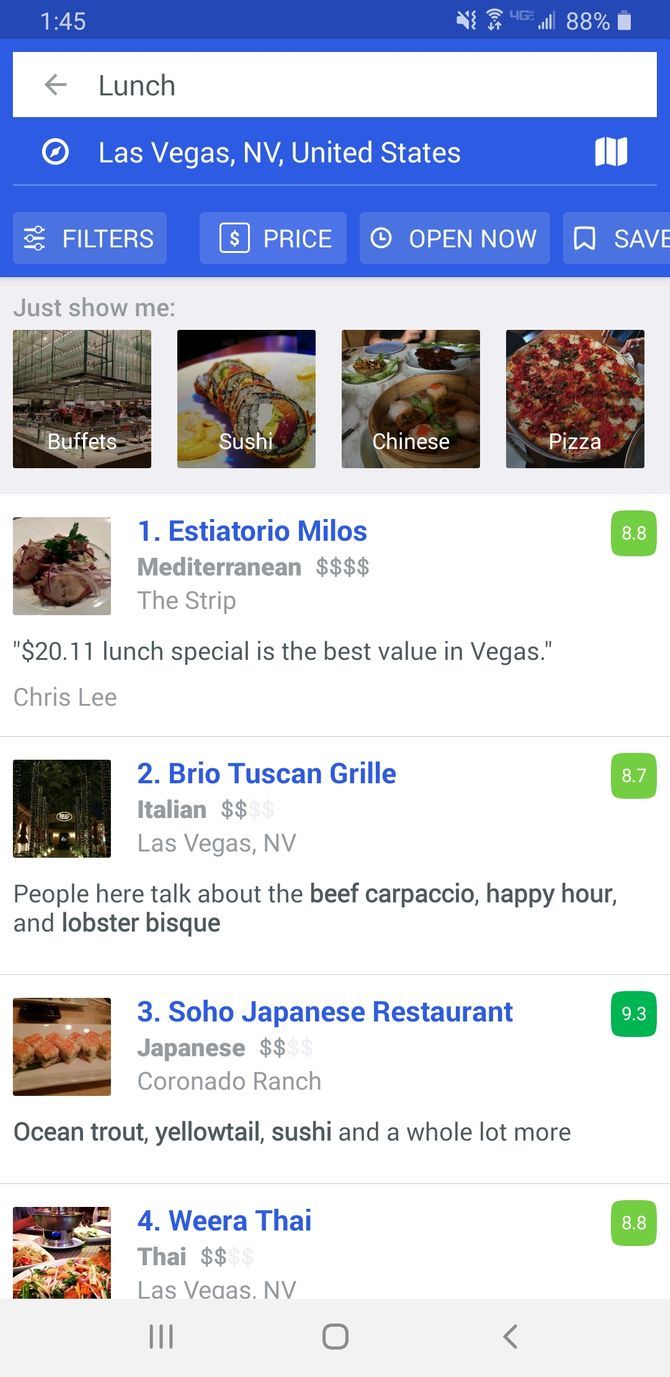The photograph is a screenshot of a mobile application displayed on a smartphone. The device's screen shows the current time as 1:45, with a signal strength of three bars and a battery life of 88%. The user is searching for lunch options. At the top of the screen, there is a white search bar featuring a back button and the search term "lunch." The location is set to Las Vegas, Nevada, USA. Below the search bar, several filter options are visible, including "price," "open now," and "save."

At the top of the results, there are categorized tabs represented by photographs, depicting different types of cuisine: buffets, sushi, Chinese food, and pizza. The first search result is "Istasiatora Milos," a Mediterranean restaurant with a four-dollar-sign price rating, and a note highlighting that their 2011 lunch special is renowned as the best value in Las Vegas. 

The second option listed is "Brio Tuscan Grill," which has a two-dollar-sign price rating. The third is "Soho Japanese Restaurant," also with a two-dollar-sign price rating. The fourth listed option is "Wiratai," which similarly has a two-dollar-sign price rating.